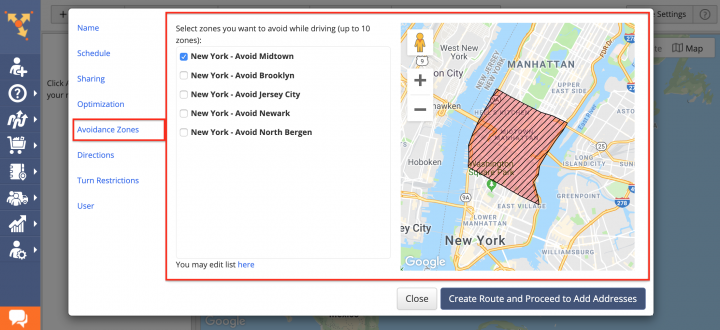The image is a horizontally rectangular screenshot displaying a map application with a pop-up window in the foreground. The pop-up has a white background and encompasses various settings for navigation customization.

On the left side of the pop-up window, rendered in blue, is a vertical list of selectable options: "Name," "Schedule," "Sharing," "Optimization," "Avoidance Zones," "Directions," "Turn Restrictions," and "User." The "Avoidance Zones" option is highlighted and outlined in red, extending this border to the right side of the pop-up, indicating the current active selection.

The detailed section for "Avoidance Zones" provides an interface for users to designate areas to avoid while driving, with a limit of up to 10 zones. The listed zones include:
- New York, Avoid Midtown
- New York, Avoid Brooklyn
- New York, Avoid Jersey City
- New York, Avoid Newark
- New York, Avoid North Bergen

The "Avoid Midtown" option has been checked, signifying its selection as an avoidance zone.

On the right side of the pop-up, there's an interactive map with a specific area visually marked by red hashing, corresponding to Midtown in New York, thus confirming the selected avoidance zone.